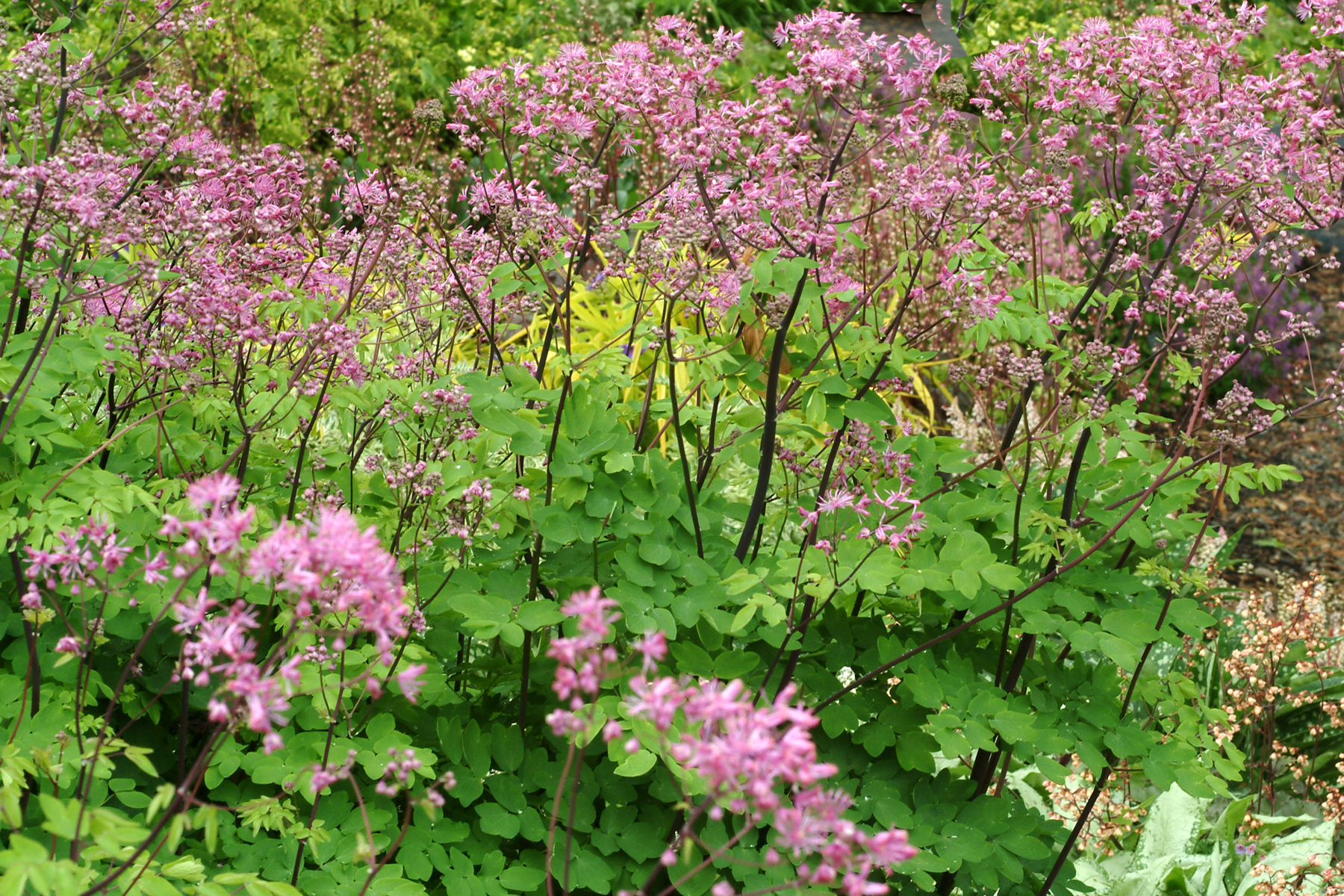This daytime photograph, likely taken in late morning or noon under a high sun, captures a lush outdoor setting along the edge of a wood or meadow. At its forefront, a densely packed patch of wildflowers dominates the scene, featuring towering stems that rise well above a bed of low bushes and green leaves. Atop these stems bloom vibrant purple flowers, similar to foxglove or lavender, with very small petals. Interspersed among the greenery are splashes of pink, as well as hints of yellow, brown, and black, adding to the diversity of colors. The flowers appear slightly shriveled, possibly nearing the end of their lifecycle. The photo, though seemingly casual and not professionally taken, skillfully frames the flowers from a side view, giving prominence to the flora without focusing on any single bloom. With no text, people, or borders present, the image exudes a natural, unmanicured beauty, suggesting a spontaneous capture by a passerby who appreciated the raw charm of the scene.